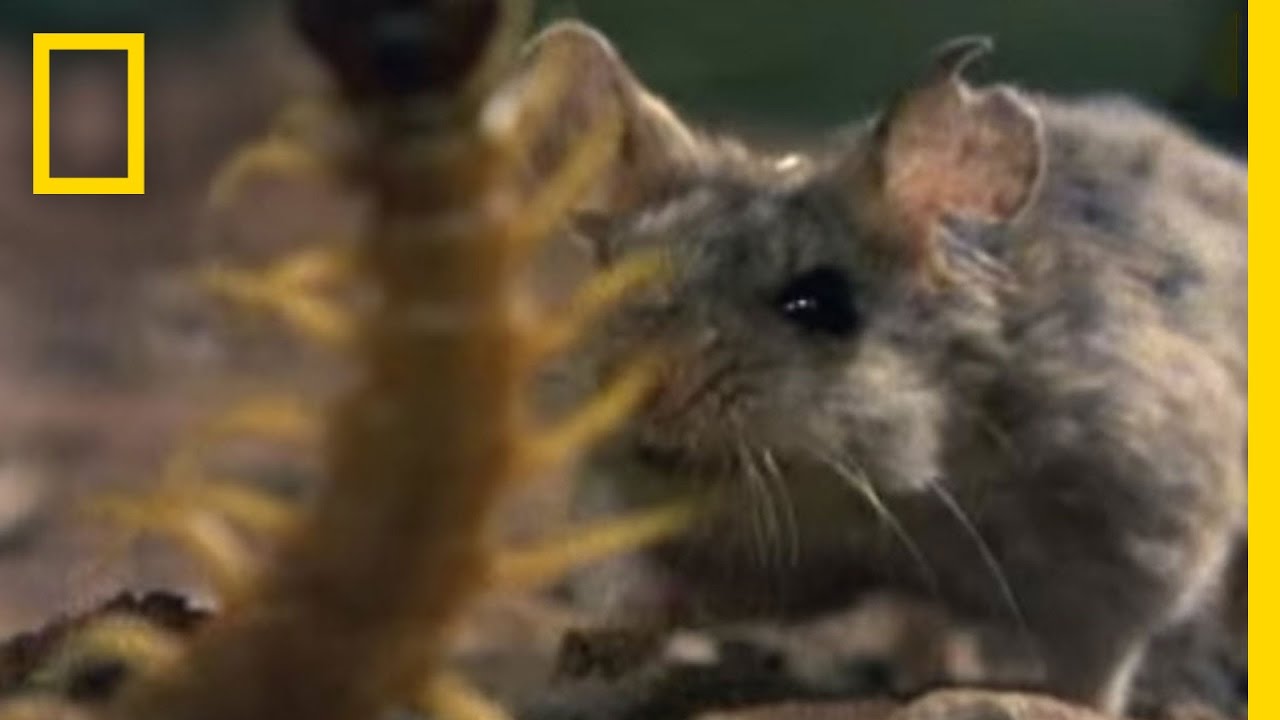This image, resembling a still from a National Geographic show, features a close-up, though blurry and grainy, of a gray mouse with very round ears, one of which has a distinctive chunk missing. The mouse, with one shiny black eye and white whiskers, stands poised with its attention focused on a giant yellow centipede, which is in front of it. The centipede has a wide brown stem with greenish-yellow spikes, adding to the tension of the scene. The photograph has a thick yellow vertical border on the right side and a yellow rectangle in the upper left corner, reminiscent of the classic National Geographic logo, emphasizing the dramatic moment of predator and prey in the wild.